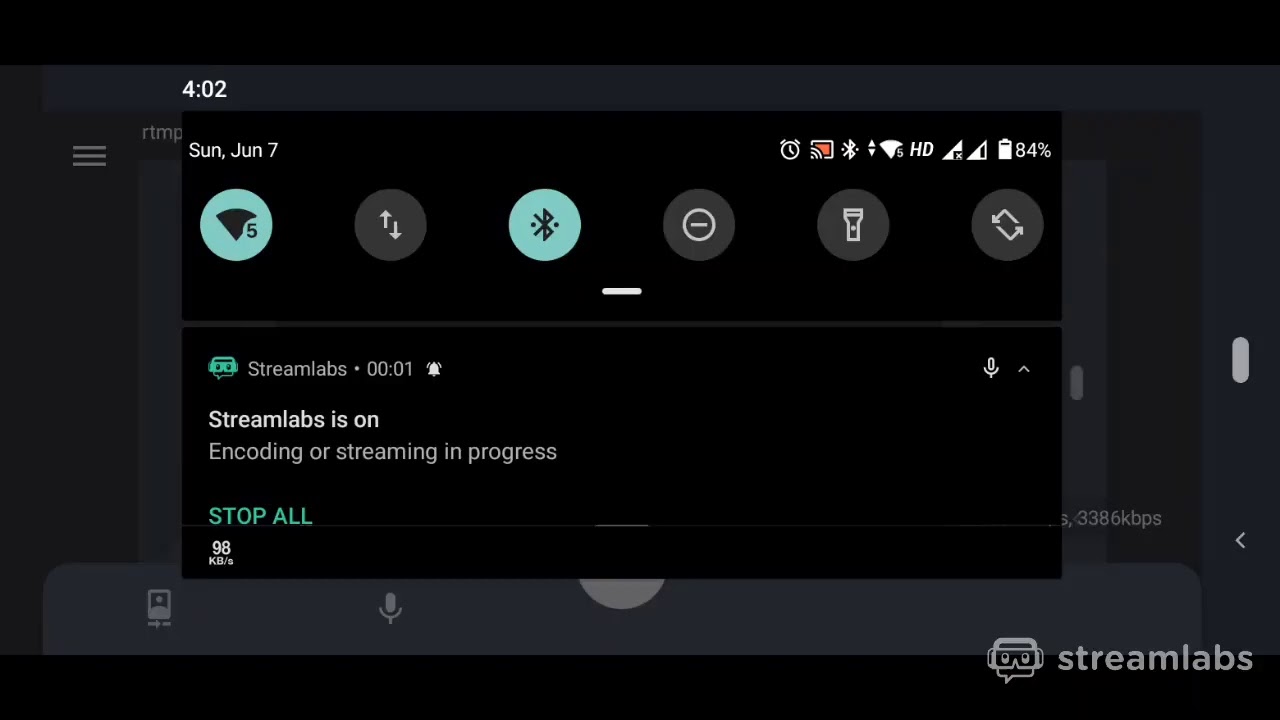A screenshot taken from a mobile phone in widescreen landscape orientation showcasing the overlay settings page of an Android device. The time displayed on the clock in the upper left corner reads 4:02, and the date is Sunday, June 7th. The upper status bar shows icons for Wi-Fi, Bluetooth, screen casting, an active alarm, and an 84% battery indicator, all signifying the device’s active functionalities. Tucked into the bottom right corner is the Streamlabs watermark featuring their distinctive logo, a chat bubble with glasses and eyes. The notification area reveals that Streamlabs is active, showing an encoding or streaming process in progress with a data rate of 98 kilobytes per second. A prominent notification indicates "Streamlabs at 00:01 - Streamlabs is on, encoding or streaming in progress," alongside a "Stop All" button, highlighting that the device is currently engaged in a streaming session.